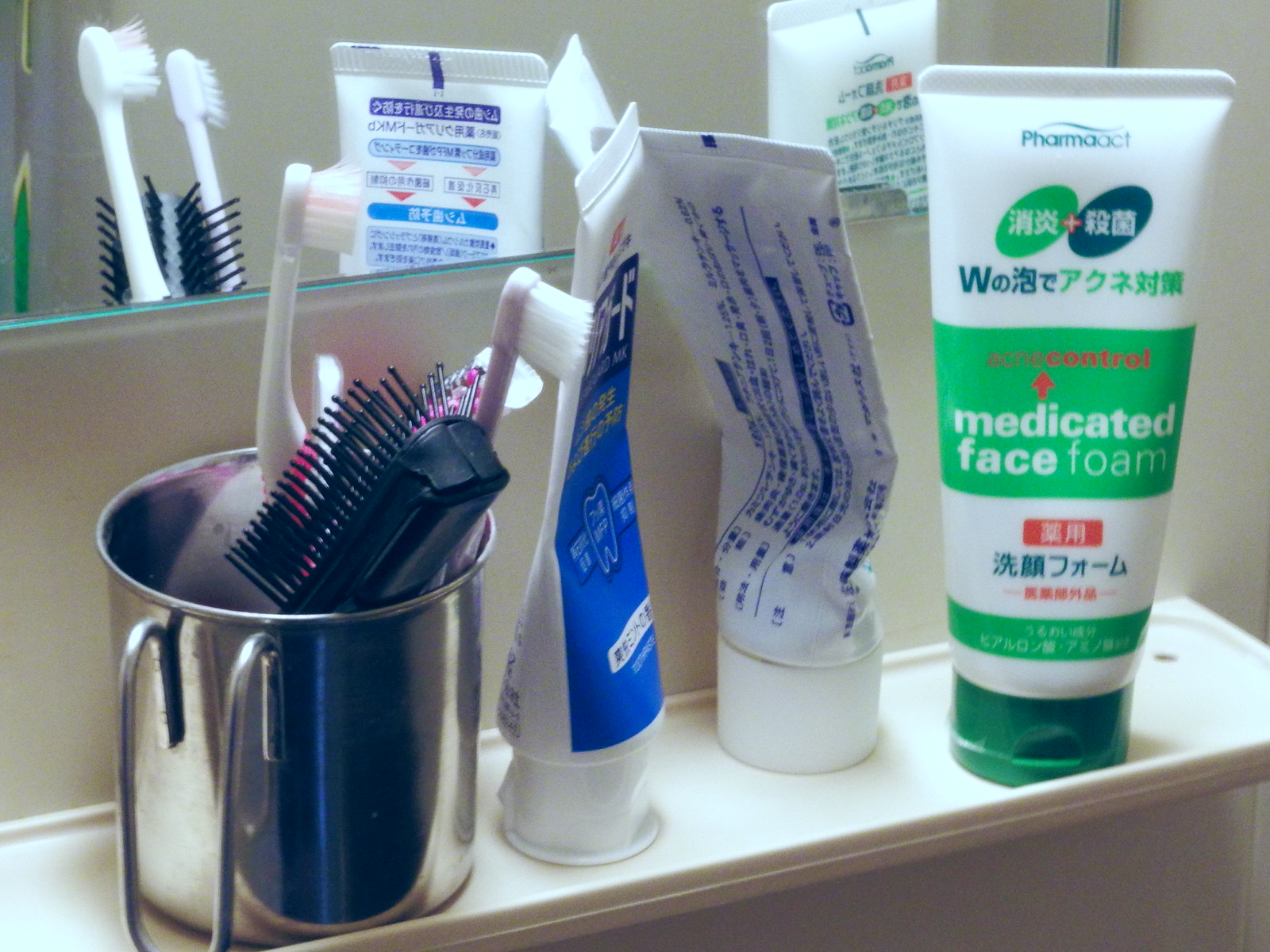This photograph depicts a well-used white plastic shelf in a bathroom, positioned directly in front of a mirror that captures the reflection of its contents. In the metallic cup, there is a black plastic hairbrush alongside two toothbrushes—one white with purple accents and the other completely white, with slightly worn bristles. The shelf prominently features three toiletry tubes: a blue and white tube of toothpaste with an image of a tooth, written in Japanese; a second tube discernible only from its back, marked by oriental script; and a green and white tube labeled "Pharma Act," adorned with light and dark green circles and Japanese writing, identified as "Medicated Face Foam." The wall behind the shelf is a light beige, complementing the orderly but clearly utilized arrangement of personal care items.